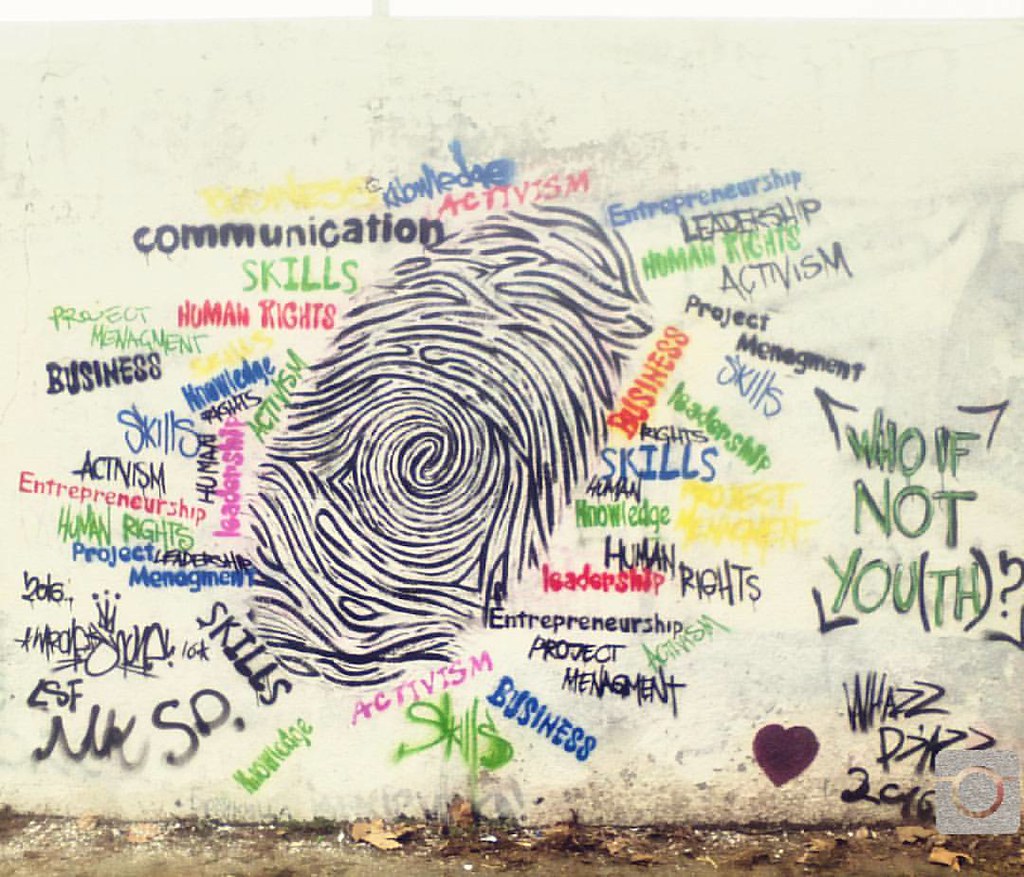The image depicts an outdoor scene featuring an old, off-white wall covered in graffiti, partially obscured by an icon on the bottom right side. Dominating the center of the wall is a large, cylindrical fingerprint, drawn in intricate black and white swirls. Surrounding this central fingerprint are various words in different colors—black, green, orange, red, blue, and yellow—forming a vibrant word cloud that includes terms like communication, activism, knowledge, leadership, business, skills, human rights, project management, and entrepreneurship. These words reflect the challenges and opportunities faced by American youth today. Below the mural, the sidewalk appears dirty brown, littered with leaves, dirt, and some rough plant life. On the side of the mural, there is a prominent message in green letters asking, "Who if not youth?" emphasizing the mural's positive reinforcement of youth empowerment.